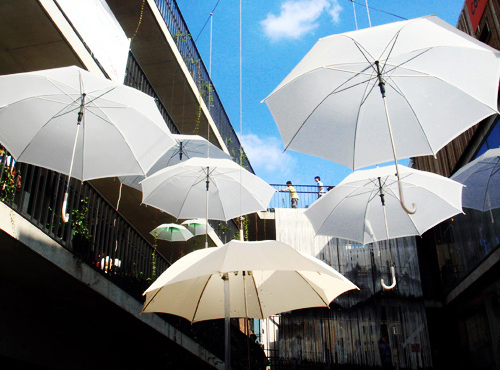This detailed photograph captures an artistic display set within a courtyard of an urban area or possibly a museum. The central focus is a series of seven white umbrellas with white handles, all opened and suspended mid-air from cables strung between two multi-level, light-colored buildings with dark wrought iron balconies. The clear blue sky, dotted with puffy white clouds, creates a picturesque backdrop, highlighting the space between the buildings. Flowering plants adorn some of the balconies, adding a touch of nature to the scene. Notably, two individuals are visible on the top balcony, observing the courtyard below. This inventive installation of umbrellas creates an intriguing and charming visual spectacle within the urban environment.